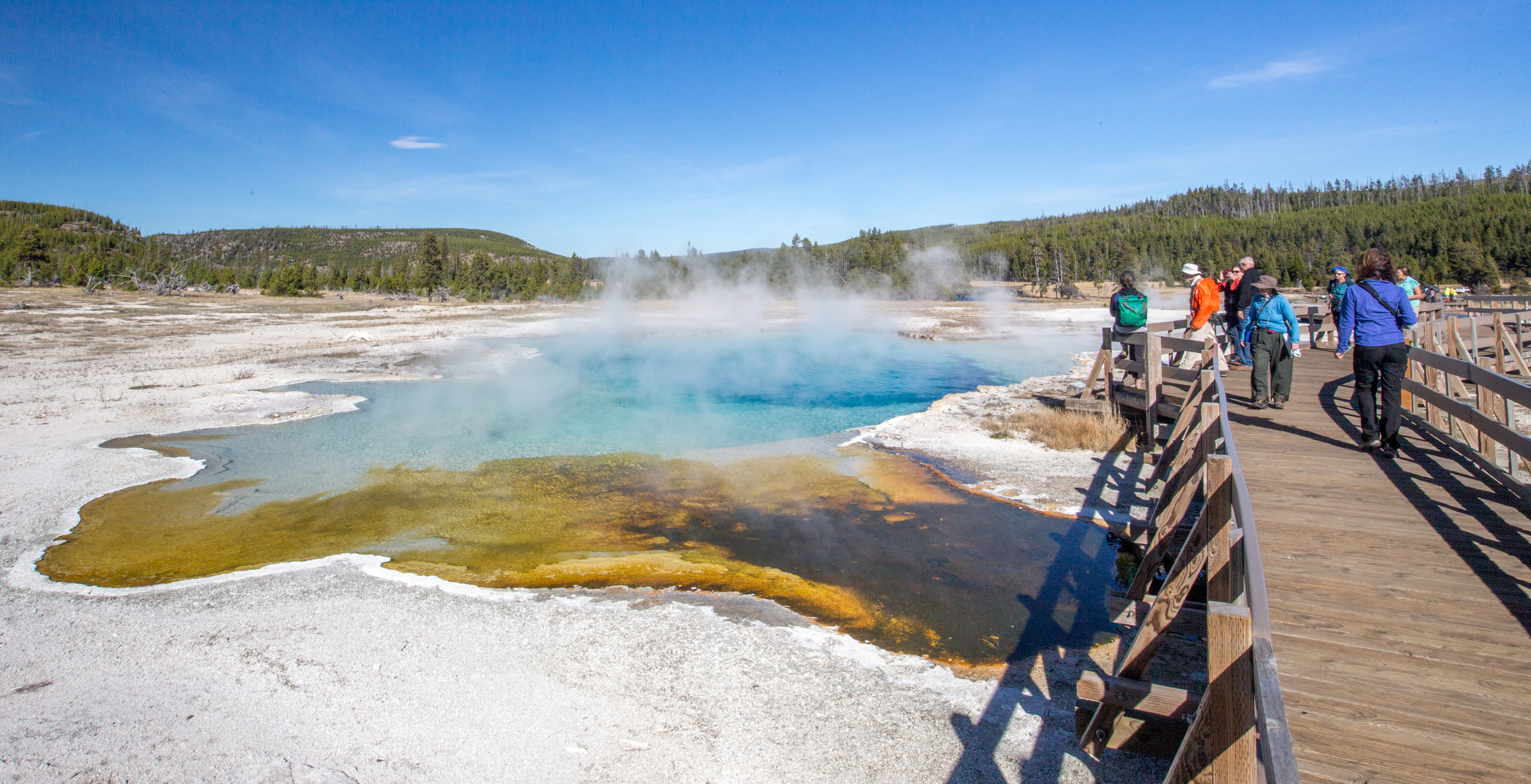This daylight photograph, taken in Yellowstone National Park, captures a stunning natural hot spring, which dominates the center to the left of the image. The hot spring shimmers with a deep blue at its center, transitioning into a grayish light blue toward its edges, where algae floats atop the water. Steam gently rises from the spring, adding to the vibrant and clear scenery. 

On the right, a wooden boardwalk lines the spring, populated by various tourists who are either walking or standing to admire the sight. The boardwalk's presence emphasizes the attraction's appeal to visitors. Surrounding the hot spring is white soil interspersed with patches of tan grass, set against a backdrop of green trees and gently rolling hills. The clear, blue sky with only sparse, thin clouds suggests the photograph was taken not during the peak of summer, yet still displays the lively hues of nature.